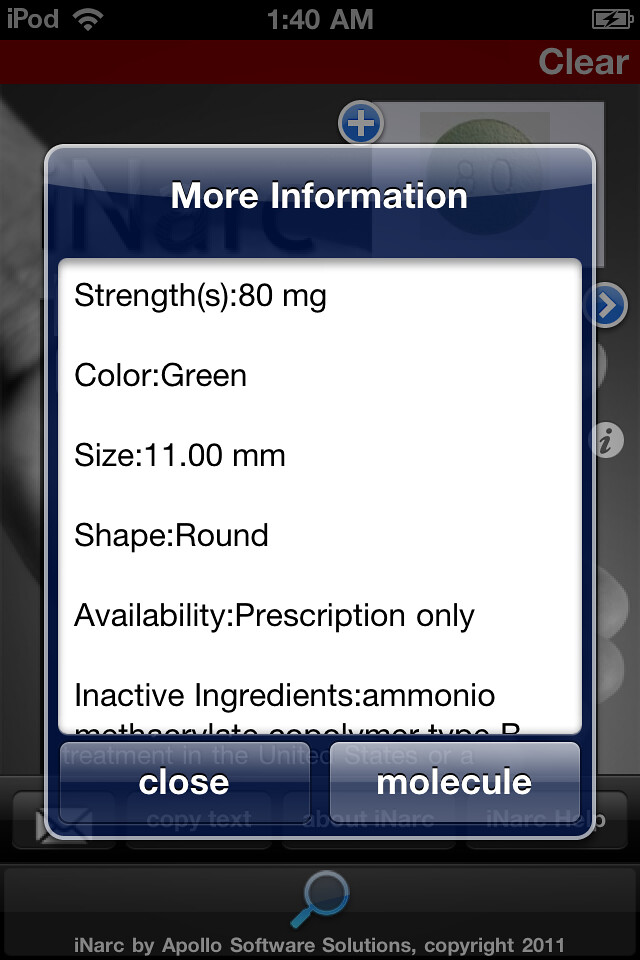This image is a detailed screenshot from an iPod, captured at 1:40 AM, as indicated by the time display at the top center of the screen. On the upper left, it says "iPod," followed by the wireless signal indicator. On the far right, there's a battery icon showing a charge. The main focus is on a pop-up information box with the heading "More Information" in white text, set against a light blue background. Below this heading, the details provided include: 

- Strength: 80 milligrams
- Color: Green
- Size: 11.00 mm
- Shape: Round
- Availability: Prescription only

The box lists inactive ingredients, beginning with "ammonio" and mentioning other compounds. The background of this screenshot reveals a partially visible program or app called "iNarco" developed by Apollo Software Solutions, as indicated by the text at the bottom: "iNarco by Apollo Software Solutions, copyright 2011." The overall color scheme includes black, gray, light blue, dark blue, white, green, and red elements, and the interface suggests the user is likely researching medication details.